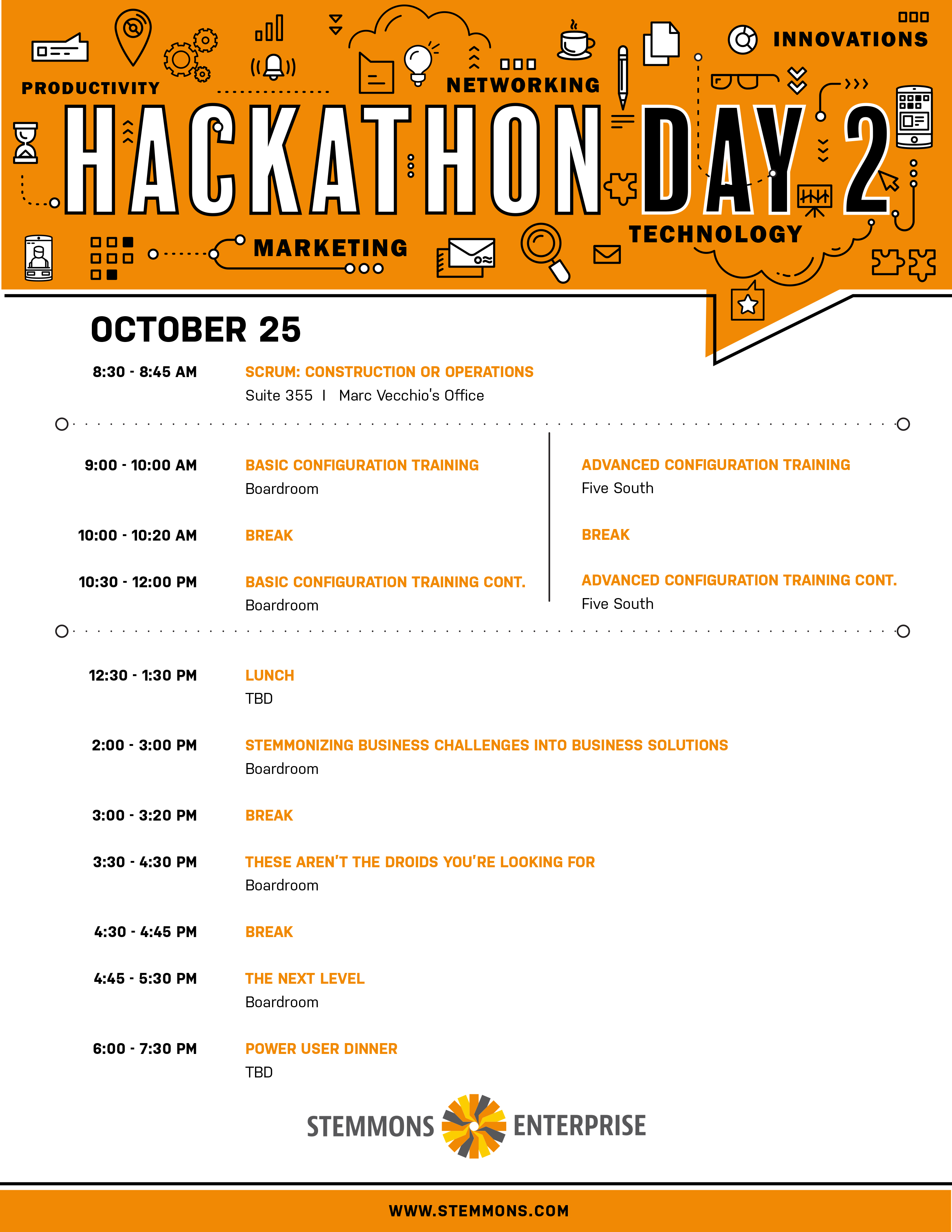The image showcases a detailed schedule for "Hackathon Day 2," predominantly colored in orange, white, and black. At the top of the image, "HACKATHON" is prominently displayed in bold, white, all-caps lettering, outlined in black, while "DAY 2" is in bold, black, all-caps lettering with a white outline. Surrounding these titles are various icons representing elements associated with computing, such as a smartphone, glasses, pencil, coffee cup, lightbulb, map icon, and hourglass. Additionally, the banner includes words like "Productivity," "Marketing," "Networking," "Technology," and "Innovations."

Below this header, the date "OCTOBER 25TH" is clearly noted, followed by an organized schedule of events that span from 8:30 AM to 7:30 PM. Each event's start time is listed in black, with details of the activities in orange, specifying their location in black text. The schedule culminates with a "Power User Dinner."

At the bottom of the schedule, the company logo of Stemmons Enterprise is displayed, featuring a pinwheel or flower design with orange, yellow, and blue petals. Below this, a horizontal black line separates the main content from an orange bar that contains the text "www.stemmons.com" in small, black, all-caps font.